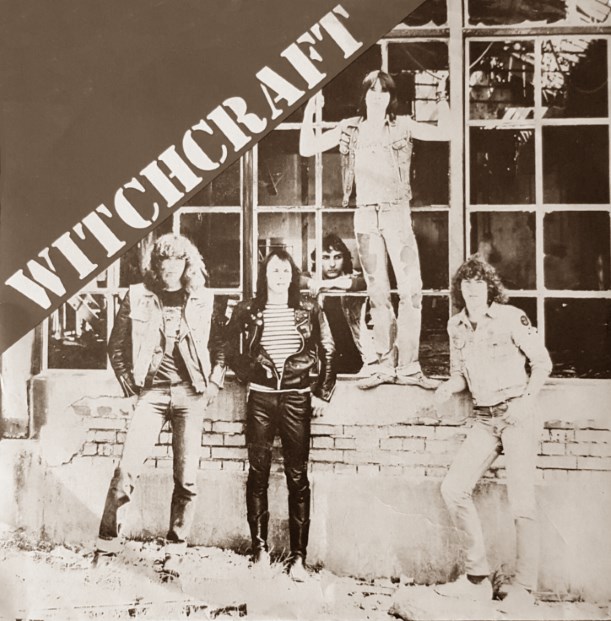In this black-and-white photograph, five young men, appearing to be members of a heavy metal rock band, are the focal point. They are standing in front of a large, possibly broken, brick wall window frame, with one of them grabbing onto the bars and another sticking his arms through it. The band members are dressed in an eclectic mix of black leather pants, a leather jacket, and tight jeans, all characterized by long, dark hair. The composition of the photo is square-shaped, suggesting it could be an album cover. Positioned diagonally in the upper left corner, white text on a black background spells out "Witchcraft," presumably the band's name. The overall scene has a gritty, outdoor urban feel, with the centered subjects and the prominent window adding to the striking visual narrative of the image.